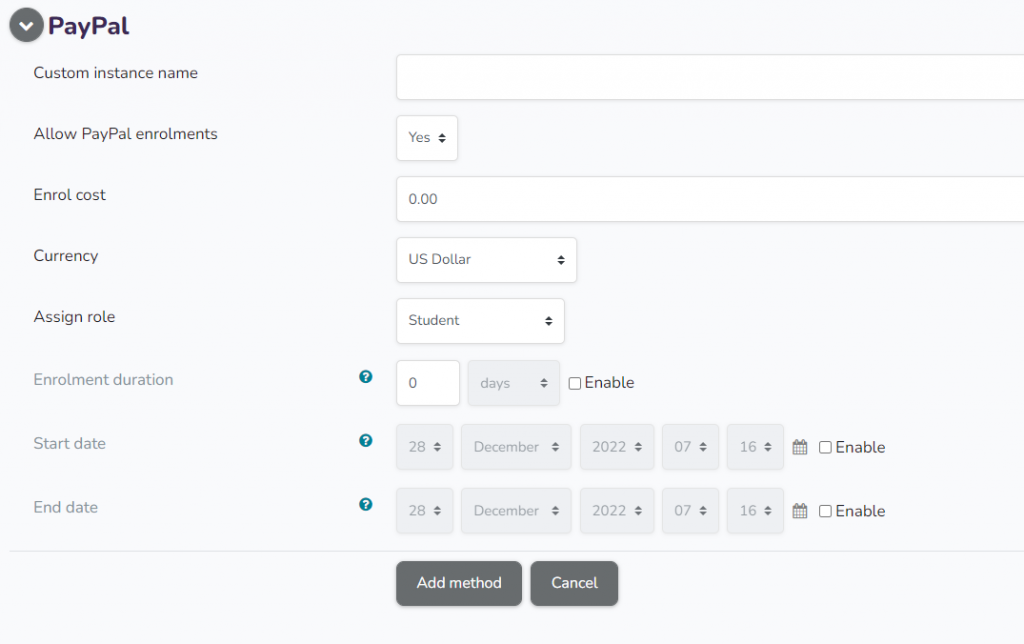The image depicts a screenshot of an older PayPal webpage, possibly from the 2010s. In the top left corner, there is the PayPal logo, which differs slightly from the current version. Below the logo is a circular icon with a white arrow inside, which appears to function as the home button.

Under the header, there are several categories displayed. The first category is labeled "Custom Instance Name." Beneath it, there is an option allowing PayPal enrollments, currently set to "Yes." The next category, "Enroll Cost," is missing an "L," and it displays a value of "00." The currency is set to US dollars.

Further down, the "Assigned Role" is set to "Student." A grayed-out option for "Enrollment Duration" is also visible, accompanied by a checkbox that is not enabled. Below this, there are fields for both the start and end dates, allowing the user to select the day, month, year, and potentially the time. However, the corresponding "Enable" buttons for these options are not activated.

At the bottom of the form, there are two gray buttons labeled "Add Method" and "Cancel."